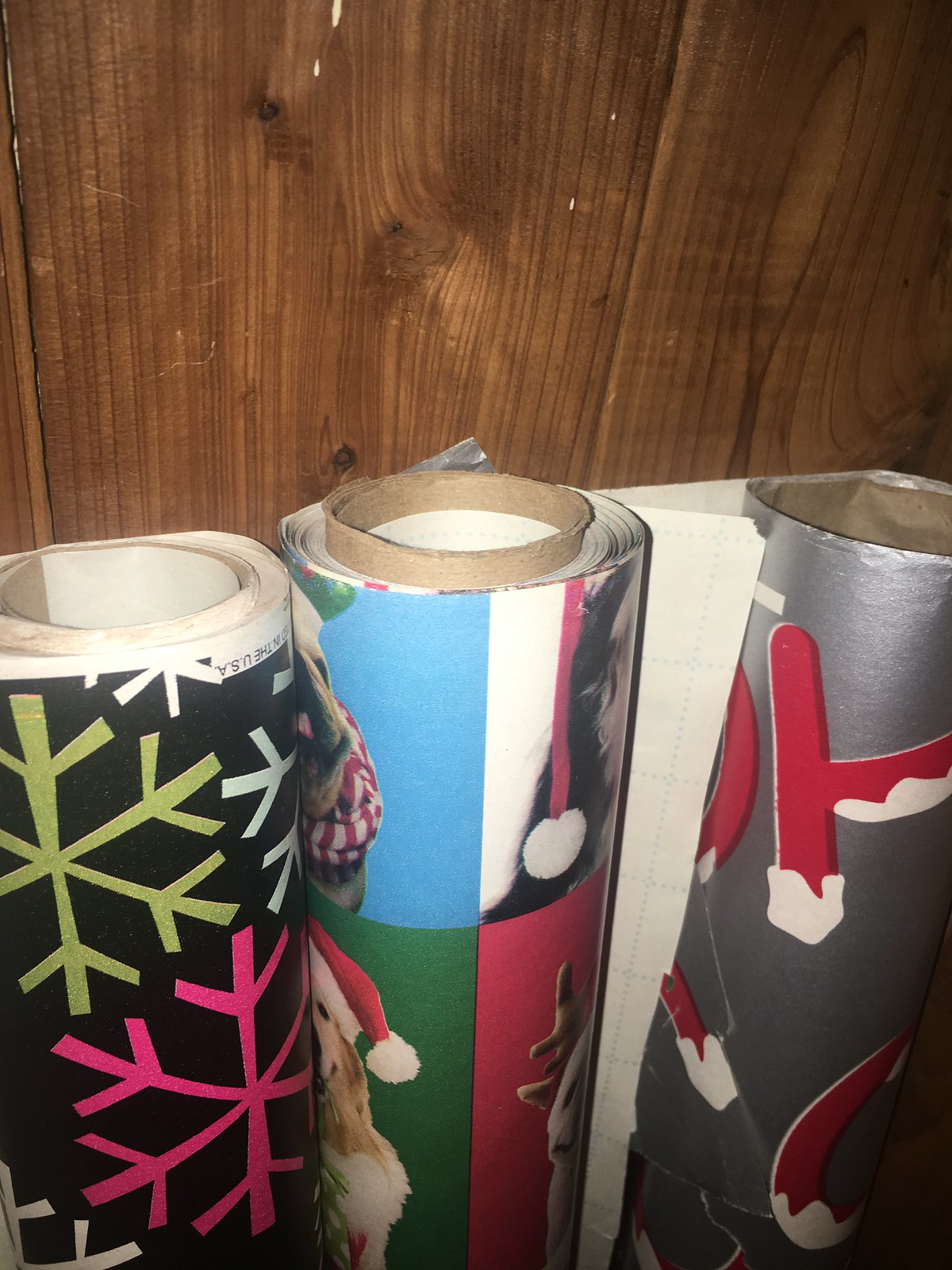The photograph depicts several rolls of Christmas-themed wrapping paper stored in a box against a wooden wall, likely within a closet. To the left, a roll features a black background adorned with snowflakes in various colors including pink. The middle roll showcases dogs wearing festive holiday attire on backgrounds of different colors. Another roll, nearly depleted, has a gray background with jolly red writing. Finally, there is a roll with a snowy design. Most rolls appear to have plenty of paper left, with the exception of the gray one. The setting appears to be a storage space for wrapping paper between Christmas seasons.